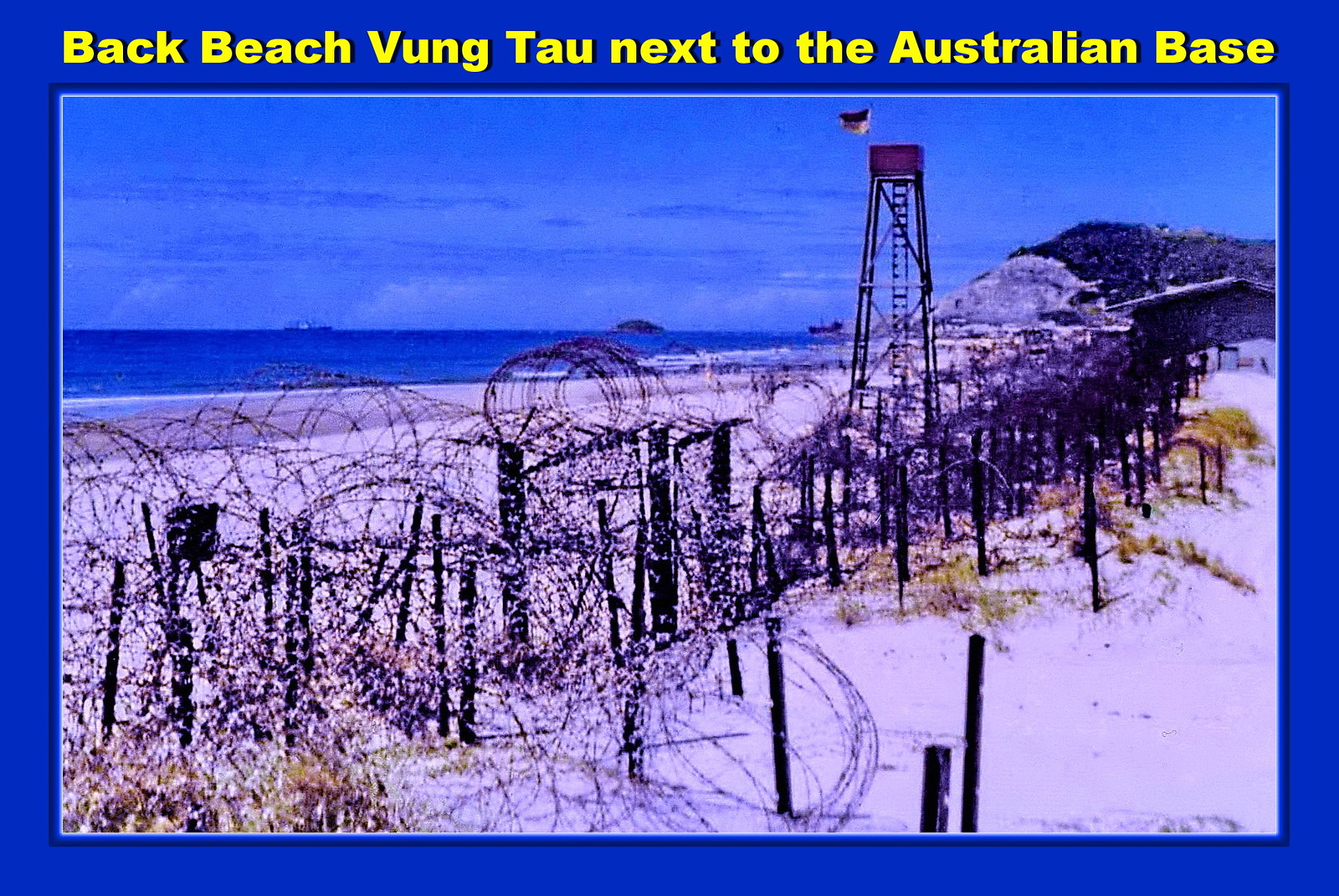This color photograph depicts a beach scene at Back Beach, Vung Tau, near the Australian base, with the title written in yellow on a blue border surrounding the image. The striking blue water dominates the left side of the photo, extending into the horizon beneath a similarly blue sky. The seashore, covered in light tan sand nearly white in color, is crisscrossed by a prominent black barbed wire fence that extends from the upper right to the lower left, spiraling back on itself. This fence, lined with wooden posts and wrapped in razor wire, segments the beach and appears to transition into what may be black trees in the grainy distance. Centrally, on the beach and water side of the barbed wire, stands a wooden lookout tower approximately two to three stories tall, featuring a ladder leading up to a platform. From the top of this platform, an American flag waves in the wind. In the background, beyond the calm expanse of blue water, a range of gray mountains is faintly visible, adding depth to the image. There is also some grass sprouting amidst the sand, adding texture to the foreground.